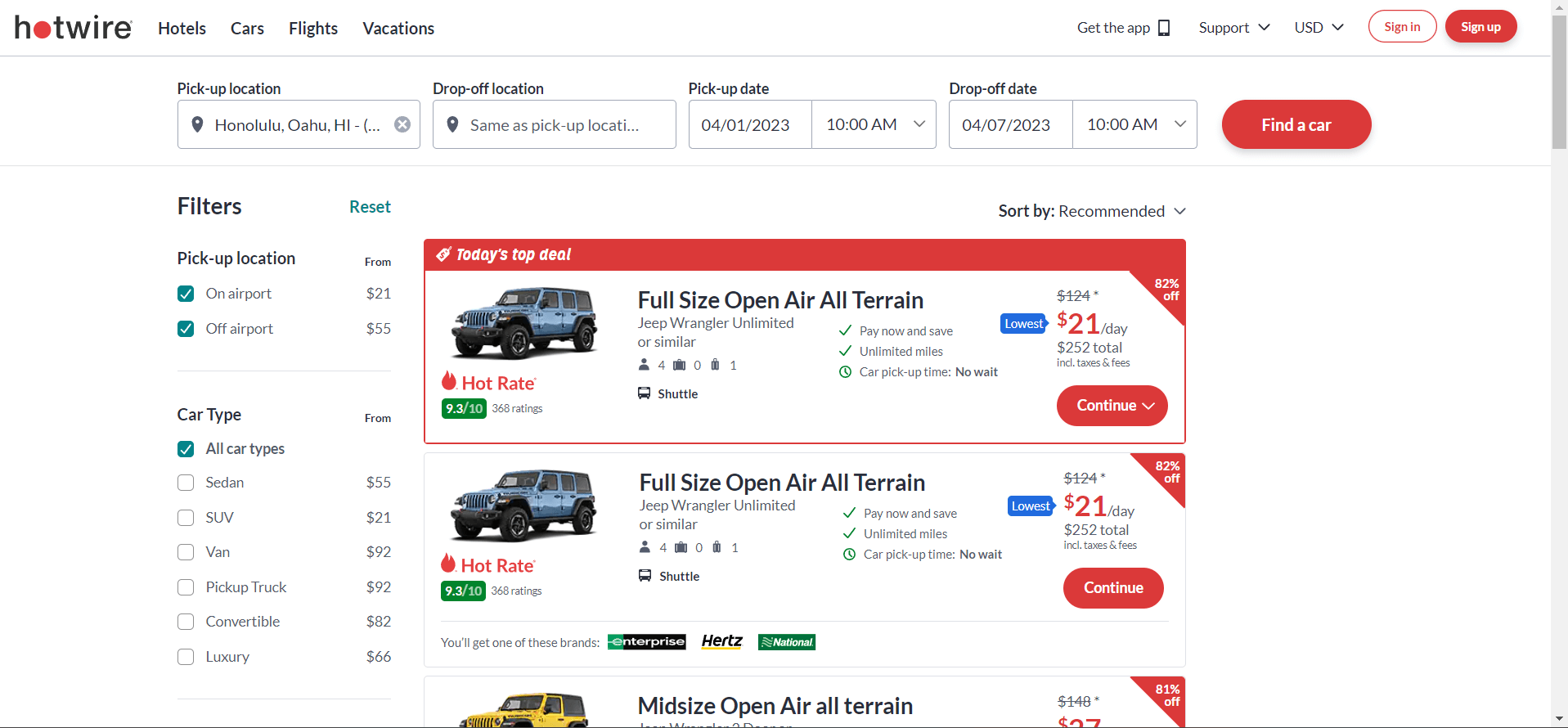This cropped screenshot of the Hotwire.com website features a predominantly white background. In the top left corner is the Hotwire logo. To the right are navigational categories in small black font: Hotels, Cars, Flights, and Vacations. On the far right, there is an option that says "Get the app" accompanied by a small cell phone icon. Next to it is the "Support" link, followed by a dropdown menu set to US dollars, and buttons for "Sign In" and "Sign Up."

Below this, centered at the top of the page, are fields for searching car rentals: a "Pickup Location" text box, a "Drop-Off Location" text box, a "Pickup Date" field with a dropdown for selecting the time, and a similar "Drop-Off Date" field with its own time dropdown. On the far right is a prominent red button labeled "Find a Car."

To the left of the page is a vertical list of filtering options. At the top left of this section, "Filters" is displayed with a blue "Reset" button beside it. There are various categories for filtering search results, including Pickup Location and Car Type.

To the right of this filtering section are three featured car listings. Each listing is marked with a red box. At the top left of each box, "Today's Top Deal" is highlighted. A photo of a Jeep Wrangler is displayed on the left side of the first listing. The middle of the box provides the vehicle's name and details, while the price is shown to the right. Each listing concludes with a red "Continue" button.